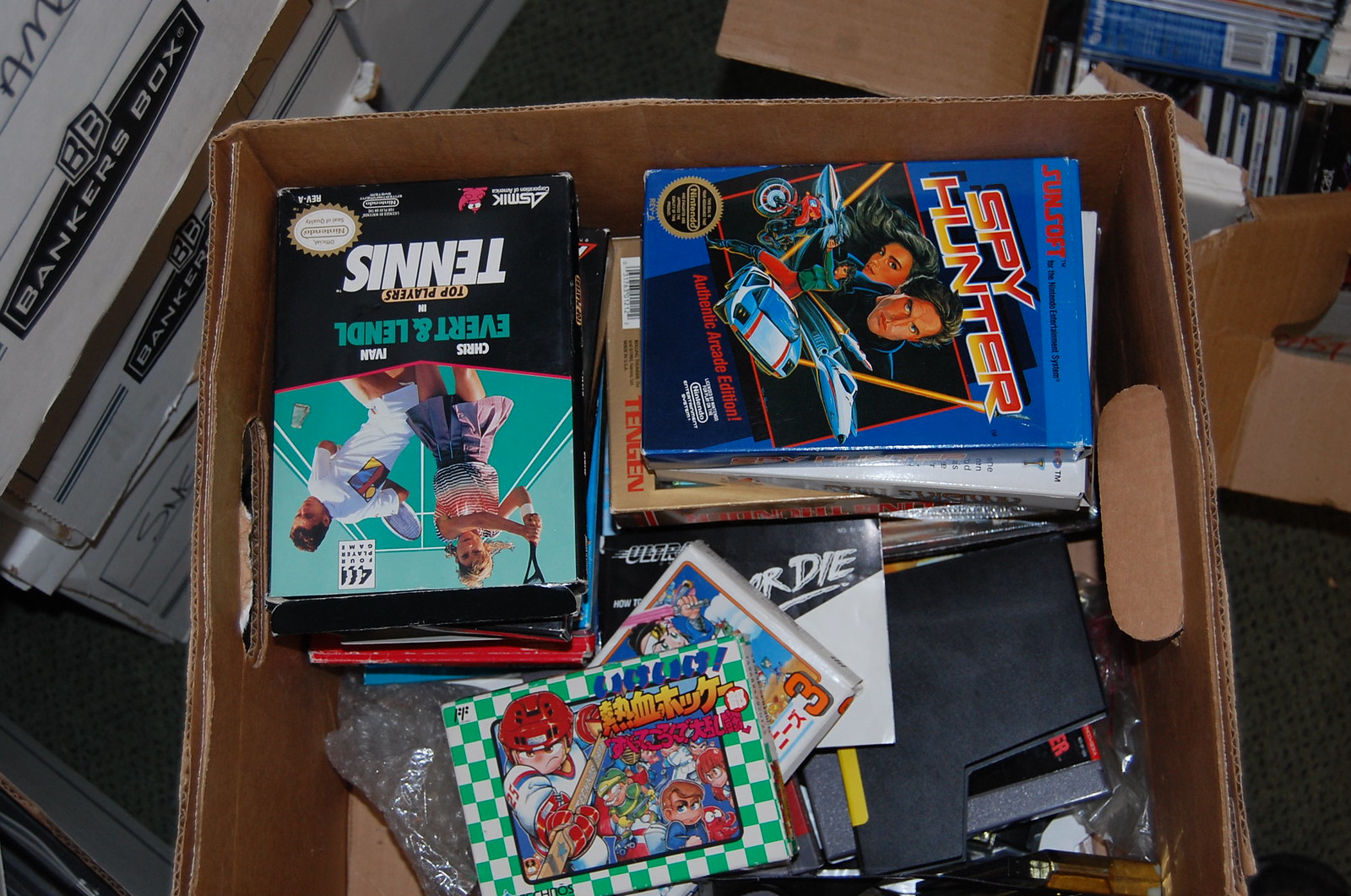This indoor photo offers a detailed top-down view of a collection of retro video games neatly organized in an open cardboard box. Dominating the image, the box is brimming with various NES and Famicom games. At the forefront, a sports game in Japanese stands out with a unique box style, possibly a hockey game. Directly next to it, an upside-down game labeled "Everet and Lindell Top Players Tennis" is distinguishable, clearly meant for the NES. In the top right corner, the royal blue box of "Spy Hunter" features prominently, its sideways orientation showcasing two women, a man, and a racing car with red stripes, complete with the label "Authentic Arcade Edition." Surrounding these games are several other NES titles, neatly stacked. In the background, partially visible boxes may contain Dreamcast or PlayStation games, possibly CDs, stacked in a hierarchical order to the left. Additionally, a white banker's box with its lid on is discernible to the left, preventing a view of its contents. The lower left corner of the main box contains a bit of bubble wrap, adding to the sense of a carefully curated collection.